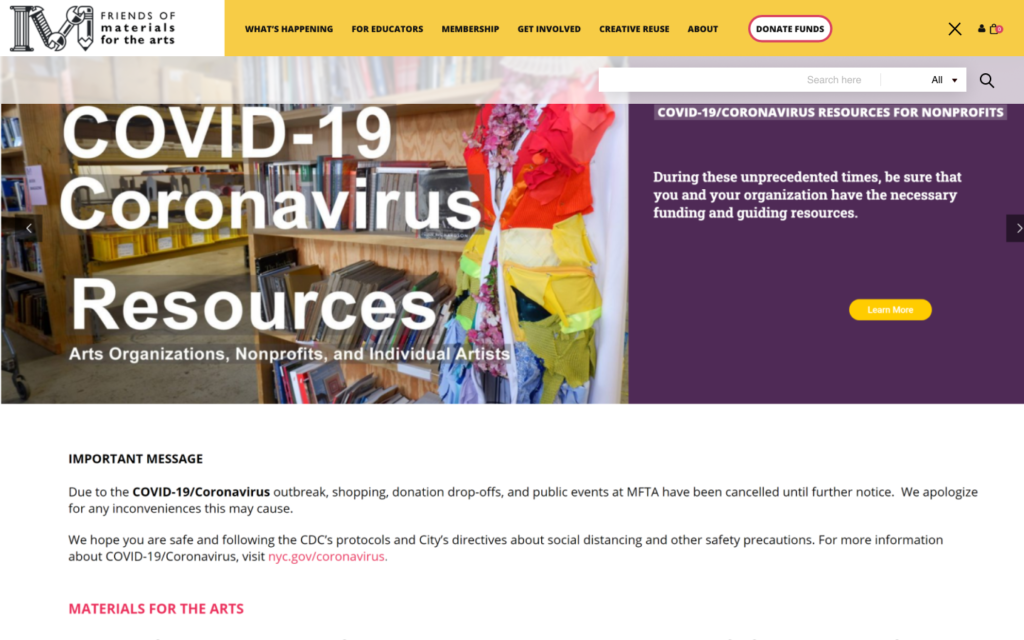This detailed caption describes a website screenshot for Friends of Materials for the Arts, highlighting the various features and information presented on the homepage:

---

A detailed screenshot of the Friends of Materials for the Arts website. At the top of the page, there are several navigation tabs labeled as follows: "What's Happening for Educators," "Membership," "Get Involved," "Creative Reuse," and "About." To the right of these tabs are buttons for "Donate Funds," an "X" button, and a shopping cart icon indicating a shop function. 

The central section of the homepage prominently displays a message titled "COVID-19/Coronavirus Resources," targeting arts organizations, nonprofits, and individual artists. It emphasizes the need for these groups to secure necessary funding and guiding resources during these unprecedented times, with an invitation to "Learn More."

At the bottom of the page, there is an important announcement noting that due to the COVID-19 outbreak, all shopping, donation drop-offs, and public events at MFTA are suspended until further notice. The notice apologizes for any inconvenience and encourages visitors to follow CDC protocols and city directives on social distancing and safety precautions. For more information, users are directed to visit nyc.gov/coronavirus.

Further down the page, the text "Materials for the Arts" overlays an artistic image created from reused materials, resembling a library bookshelf filled with books and other items.